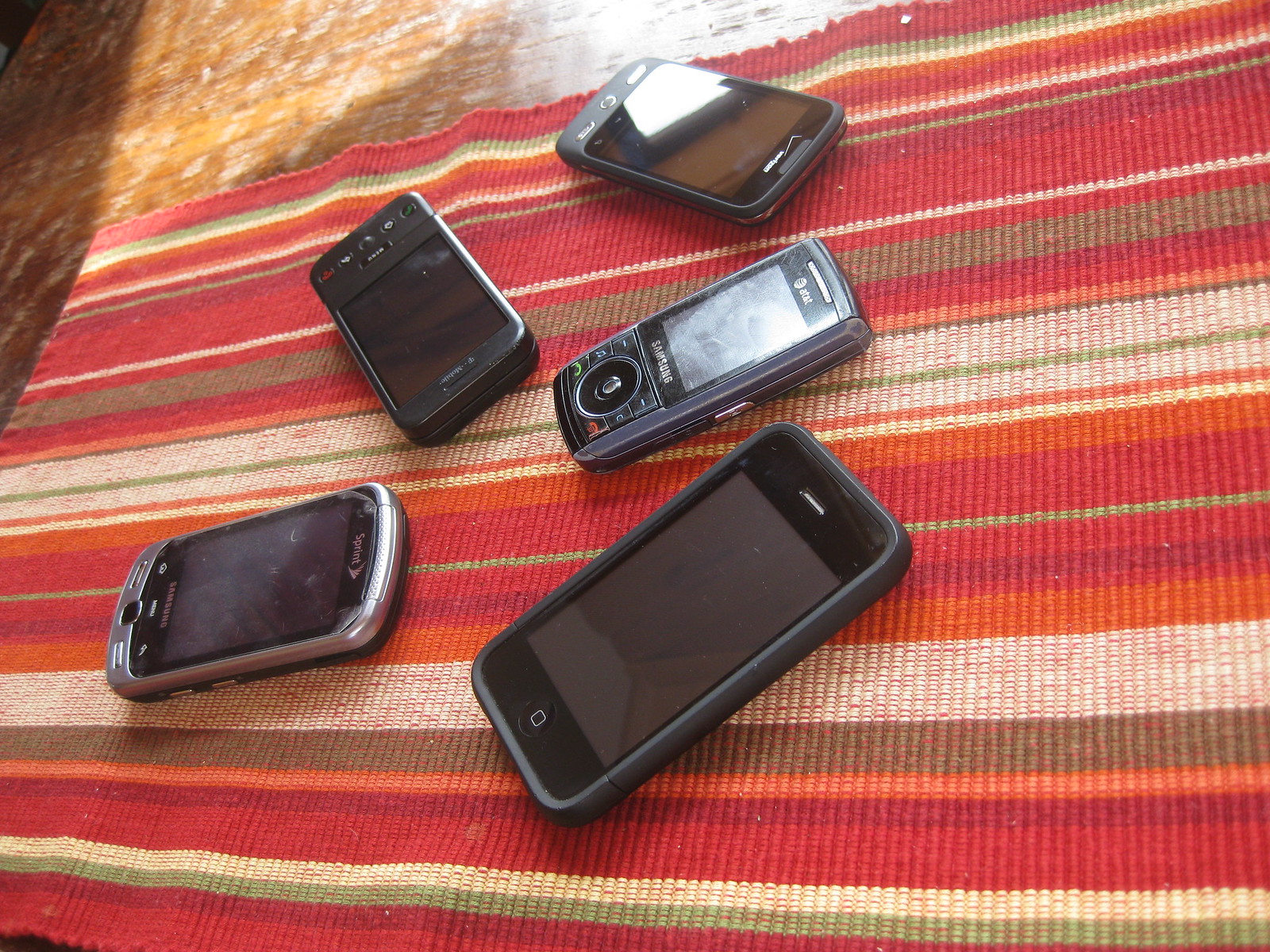This landscape-format photograph showcases five assorted, old-fashioned mobile phones laid out on a striped rug. The rug features vertical stripes in red, light green, off-white, orange, and brown, and it sits atop a reflective wooden or laminate floor. The phones, with casings in various shades of black, dull silver, and dark gray, show signs of wear with smudges and scratches on their screens. Among the four smartphones is an older model "clicky" Samsung phone with a smaller screen. The poorly taken photo highlights the nostalgic, used nature of these devices strewn across the striped rug.